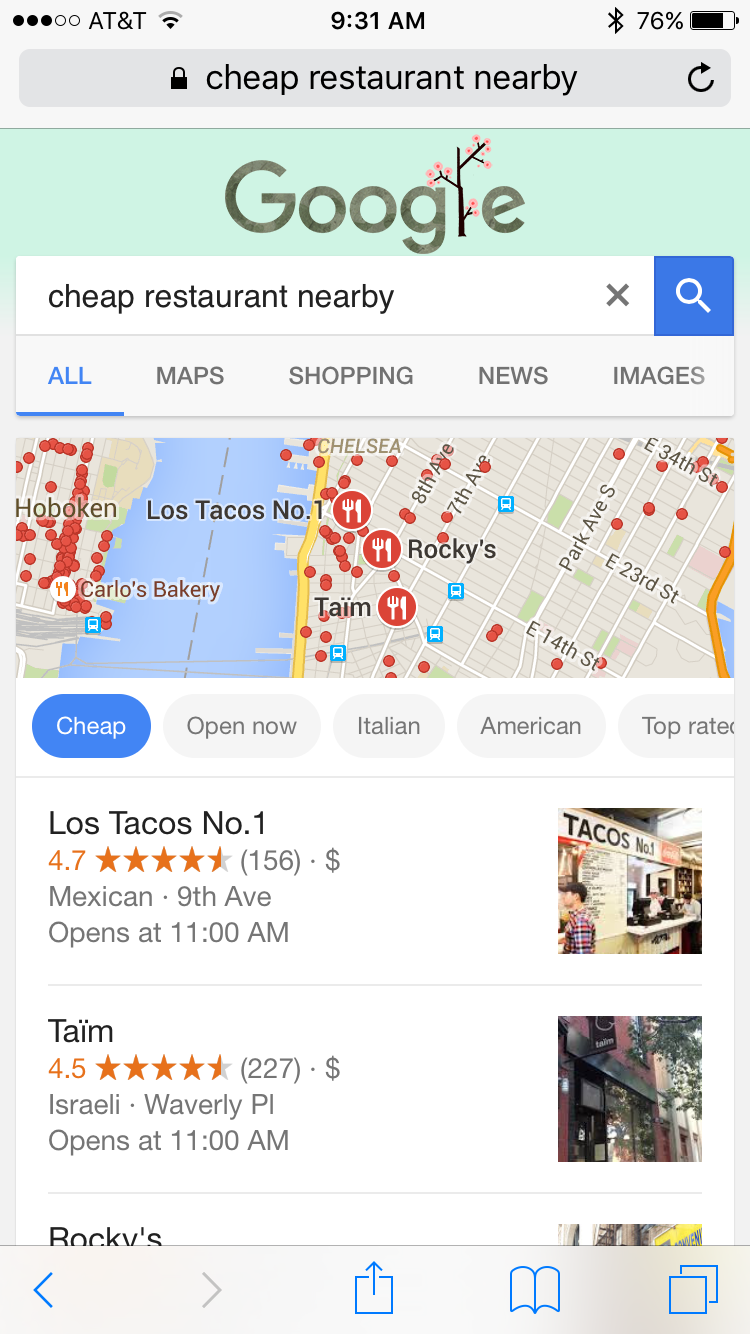The image is a screenshot taken from a smartphone, specifically using the Safari browser, displaying search results for "cheap restaurants nearby" on Google. The timestamp on the phone reads 9:31 AM, indicated in the top center of the screen. 

In the top-right corner, the battery icon shows it is nearly full with a 76% charge remaining, accompanied by a black-colored Bluetooth symbol. To the left, the top-left corner displays a cellular signal strength indicator with three black bars and two empty ones, likely representing a moderate connection. This is followed by "AT&T" and a Wi-Fi symbol with only two bars filled.

The main content of the screenshot is centered around the Google search results, showing three restaurant listings. The first result is "Los Tacos No. 1," boasting a high rating of 4.7 stars. The second entry, labeled "Time," holds a 4.5-star rating. The third listing, partially obscured but identifiable as "Rockies," is barely visible at the bottom of the screen.